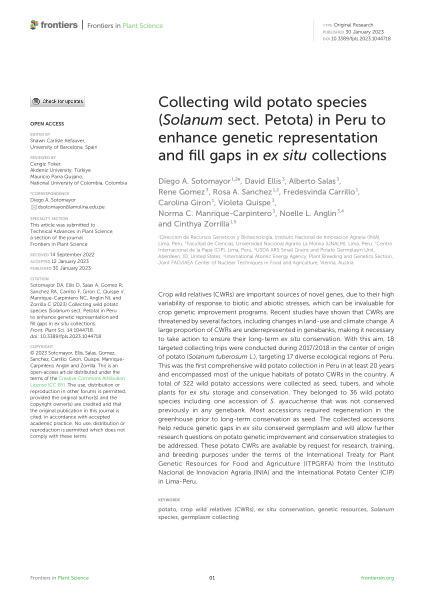The image depicts a black and white page of text, which appears to be an article from a publication titled "Frontiers in Plant Science." The top left of the page features the word "frontiers" prominently in bold lowercase letters, followed by the title of the article in slightly blurry but readable dark gray font: "Collecting Wild Potato Species (Solanum Sect. Potato) in Peru to Enhance Genetic Representation and Fill Gaps in Ex Situ Collections." The text also mentions a list of authors, including Diego A. Santo Mayor, David Ellis, Alberto Salas, Rene Gomez, Rose A. Sanchez, Fred Swinda Carrillo, Carolina Guyroin, and Violeta Quispis. Despite the difficult-to-read font, the title and context suggest the article discusses the collection and genetic modification of wild potato species to improve genetic diversity and address gaps in existing ex-situ collections. The right-hand side of the page labels the article as "original research."